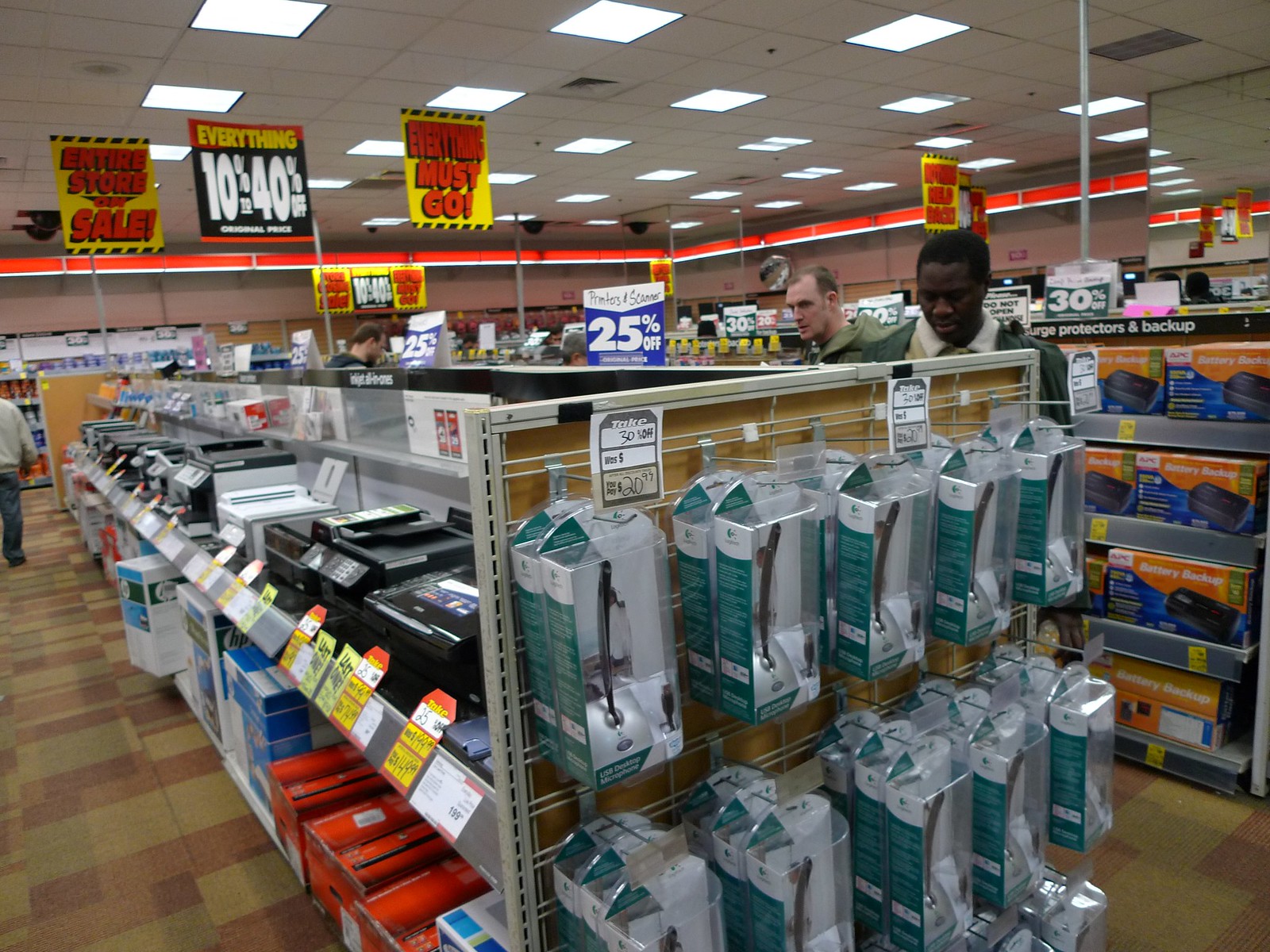The image depicts a bustling aisle in a department store, reminiscent of electronics sections in stores like Fry's or Target, although no specific store logos are visible. The foreground prominently features a shelving unit displaying a variety of tech products. On the top shelf, an array of printers is showcased, predominantly black with a few in light gray or white. Below the printers, multiple boxes are arranged; these include distinctive orange boxes and HP brand boxes that are white, blue, and green. Additionally, teal and white plastic packages containing thin, upright items are visible.

In the foreground, attached to the shelving unit, plastic boxes filled with cords can be seen. The aisle also contains numerous sale signs hanging from the ceiling. Three bright yellow signs with red print declare, "Entire Store Sale - Everything Must Go." Another sign with a black background displays "Everything" in yellow and "10% to 40% Off" in white. A blue sign indicates "25% Off" in white lettering.

Multiple people populate the scene. On the left, a black man and a white man are examining items on the middle shelves. To the right, in the adjacent aisle, several other people are visible. The floor is carpeted in a pattern of small squares and rectangles, further indicating a detailed and busy retail environment.